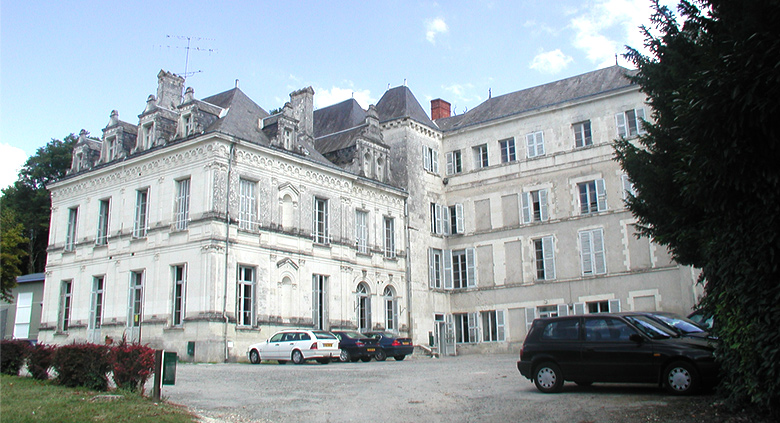The image depicts a stately manor that exudes an old European, possibly parliamentary, architectural style. The manor is primarily constructed from off-white brick or a similar hard substance and features two main sections. The left side is a two-story structure with an attic, while the right side is taller, standing at four stories. Both sections are interconnected, forming an L-shaped design. The building has a gray roof and a red chimney protruding from the back, accompanied by an antenna and some wires.

In front of the manor lies a gray parking lot with approximately five cars parked. To the left of the building, a small grassy area is adorned with red shrubs and a trash bin. Additional foliage, including larger bushes and decorative shrubs, can be seen in the foreground, some of which have a reddish hue. The setting is captured on a clear, blue-sky day with a few white clouds scattered above. Trees frame the manor on both the left and right sides, adding to the picturesque scene. The overall impression of the manor suggests a blend of historical elegance and functional design, reminiscent of a modern castle or a grand hotel.